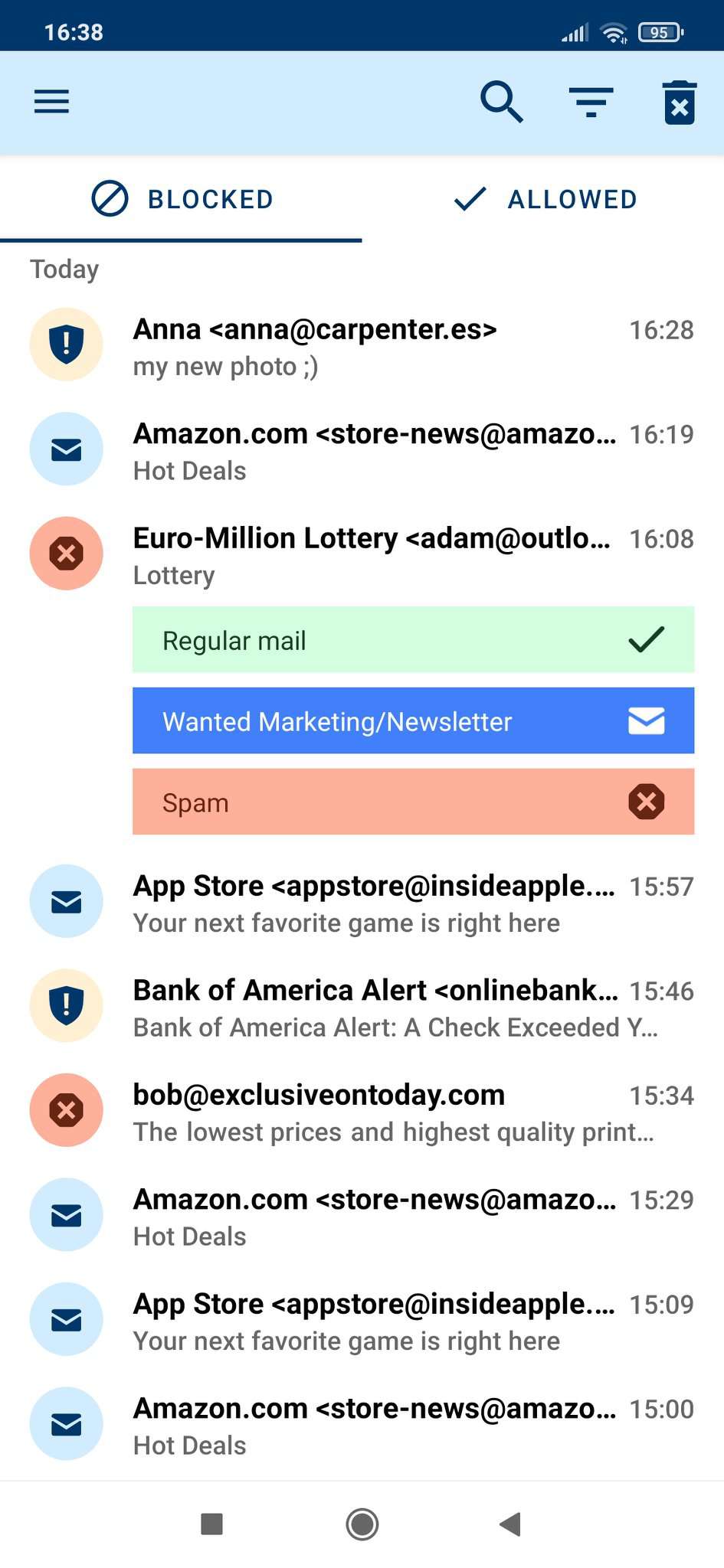A screenshot of a smartphone's messaging app interface showcasing a series of actions taken to filter messages as either allowed or blocked. At the top of the screen, the battery indicator and network connectivity bars are visible, confirming it's a mobile device. Directly beneath this, a light blue bar features several icons including a delete icon, a search icon, and an icon for altering the page's layout.

Below this bar, a chronological list of message transactions is displayed. Each entry clearly indicates whether the message was permitted or flagged as spam. For example, a message from "Anna" with the subject "my new photo 😊" is allowed, followed by an unblocked message from the "Amazon store." The first blocked message appears with a red circle containing an 'X,' labeled "Euro Million Lottery," accompanied by promotional text about the lottery.

This visual list helps the user differentiate between safe and suspicious messages, enhancing their ability to manage their inbox effectively.